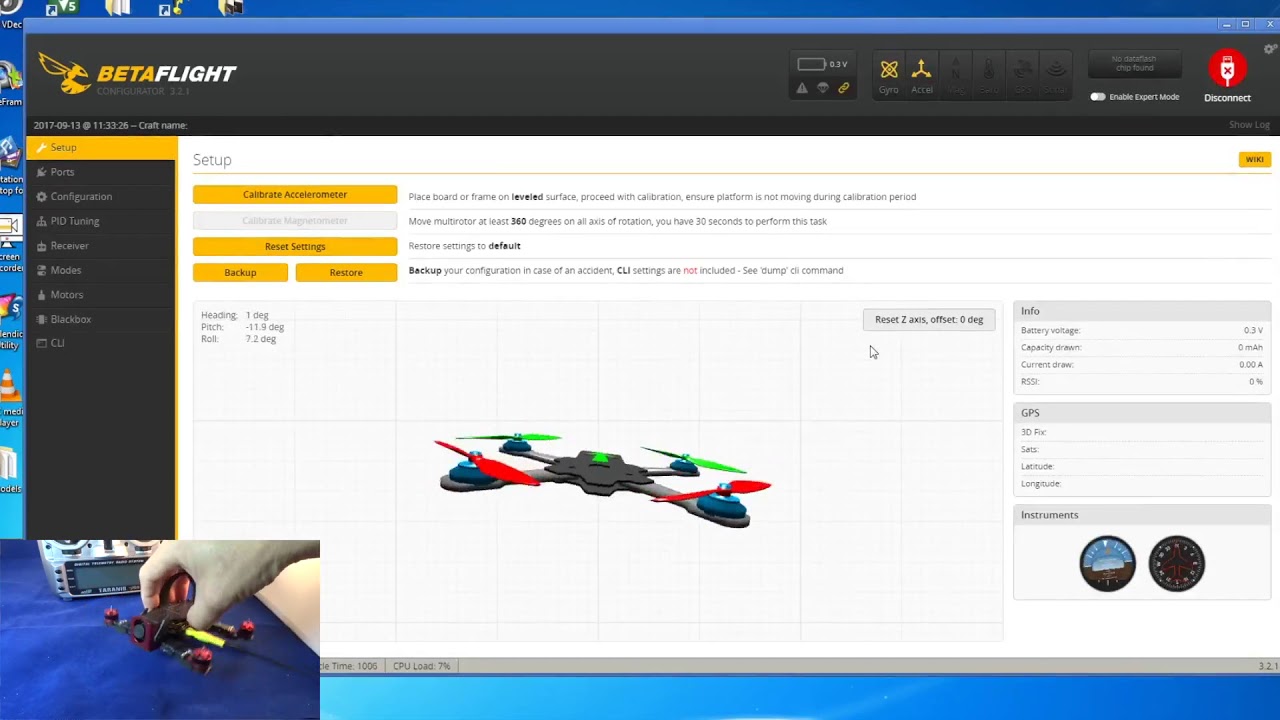This image is a detailed screenshot from the Betaflight software interface, showcasing various features and settings used for configuring drones. 

At the top of the interface, a blue header is prominently displayed, followed by a black sub-header featuring the Betaflight icon. To the right of the Betaflight icon, there are several selection buttons, which are unspecified in this description. The sub-header ends with a "disconnect" option highlighted within a bright red circle. 

On the far left side of the interface, a vertical menu lists multiple options: Setup, Ports, Configuration, PID Tuning, Receiver, Modes, Mirrors, Black Box, and CU. 

Within the main section titled "Setup," a large white triangle is positioned at the top, below which several yellow informational rectangles are displayed. One such rectangle instructs users to "Calibrate Accelerometer," advising to "Place board or frame on leveled surface" and "Ensure platform is not moving during calibration period." Additionally, there is a grayed-out button next to the instruction. Another informative yellow rectangle prompts to "Move multicopter at least 360° progressing on all axes of rotation" within a 30-second timeframe. Another gold rectangle offers the option to "Reset Settings" and "Restore Settings to Default." Adjacent to this, two more yellow rectangles labeled "Backup" and "Restore" direct users to backup their configuration to avoid accidental loss, noting that CLI settings are excluded and referring users to a specific dump command for further details.

A large box containing a faintly printed graph occupies the center of the interface. Located in the upper left-hand corner of the graph, specific readings are displayed: Heading: 1 degree, Pitch: -11.9 degrees, and Roll: 7.3 degrees. A multicolored drone image (featuring red, blue, green, and black) is centered within the graph box. 

On the right-hand side, an additional menu provides information on battery statistics and GPS data. The top section lists Info, Battery Voltage, Capacity, Current Draw, and RSD. Under the GPS section, it notes a "3D Fix" and provides fields for Latitude and Longitude. The bottom part of this section appears to contain an image of two gauges or dials, labeled as Instruments.

This comprehensive screenshot offers a detailed view of the Betaflight software, essential for drone enthusiasts who require precise control and configuration options for their devices.